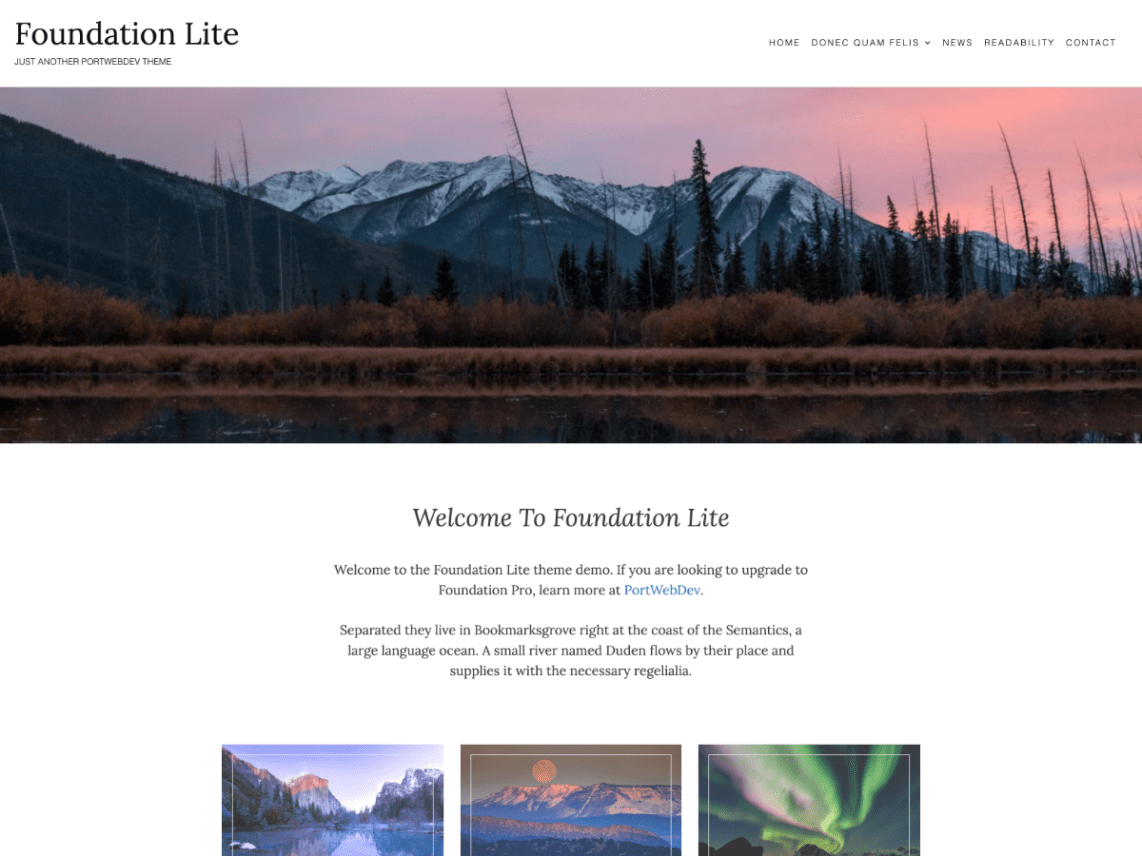**Caption:**

This image is a screenshot of a web design theme named "Foundation Light." Dominated by a pristine white background, the design prominently features a large header block at the top. Above the header block, the text reads "Foundation Light" followed by "just another something theme." Unfortunately, one word is unreadable. In the top right-hand corner, a navigation bar displays links titled "Home," "News," "Readability," and "Contact."

The expansive header bar showcases a picturesque landscape, capturing either a sunrise or sunset over snow-covered mountains with a serene lake in the foreground. The palette consists of various hues, including pink, peach, mauve, grey, and hints of brown. 

Centrally located below the header image, the text in bold announces: "Welcome to Foundation Light," followed by "Welcome to the Foundation Light theme demo. If you are looking to upgrade to Foundation Pro, learn more at PortWebDev," with "PortWebDev" highlighted in blue, indicating it is a clickable link.

Further down, the narrative continues with a whimsical description: "Separated. They live in Bookmarks Grove right at the coast of the Semantics, a large language ocean. A small river named Duden flows by their place and supplies it with the necessary regalia."

Beneath this text are three small thumbnail images of nature, aligned horizontally. The left thumbnail portrays a river beneath a sky tinged with the early morning or late evening blue. The central thumbnail captures a large moon rising over a mountain. The right thumbnail features the breathtaking display of the Northern Lights.